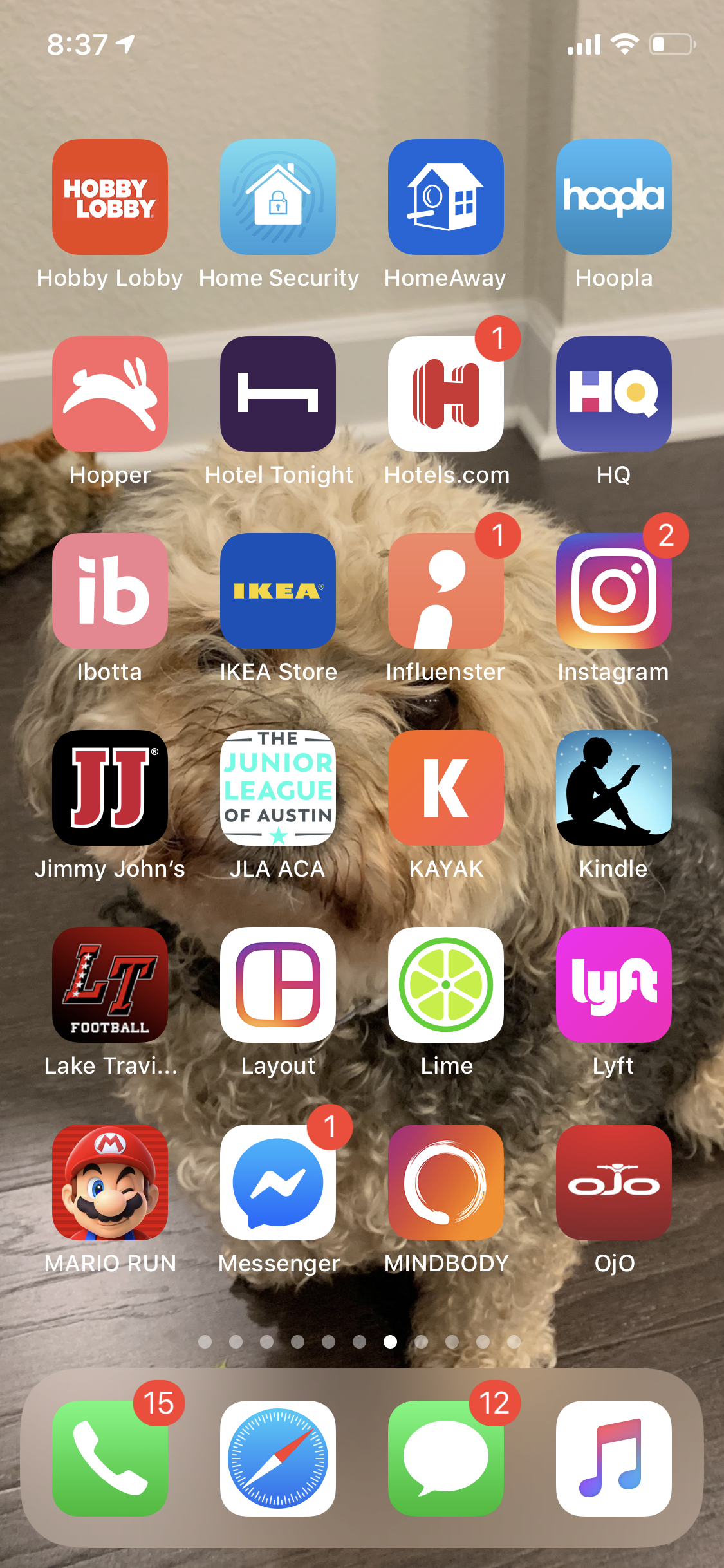This is a detailed screenshot of a smartphone home screen, showcasing various elements in a structured layout. The background image features a small, curly-haired dog with a mix of dark and light brown fur, floppy long ears, a fuzzy nose, black eyes, and fluffy bits of fur atop its head. The dog is positioned against a backdrop of a white wall and dark wood floor.

Overlaying this background image are a series of app icons arranged in a grid format. There are six complete rows of four app icons each, followed by a seventh row that is encased in a slightly transparent rectangle, allowing a faint glimpse of the background photo to show through.

Each app icon is uniquely colored and adorned with distinct symbols or logos. Among them, there is an orange square featuring a cartoon bunny, a blue square with the word "IKEA," and a pink square with a letter "K." The icons are assorted in various other colors, including green and white.

The seventh row, within the transparent rectangle, contains four specific app icons: a green square with a phone symbol, a white square with a compass symbol, another green square with a message bubble symbol, and a white square with a music note symbol. Notably, two of the green squares have a small red circle in the top-right corner, indicating notifications, each marked with a number inside.

Above the transparent rectangle, there is a set of small dots, one of which is illuminated in white, signifying the current page of the home screen. Finally, above these dots are the rows of four app icons extending up to the top of the screen.